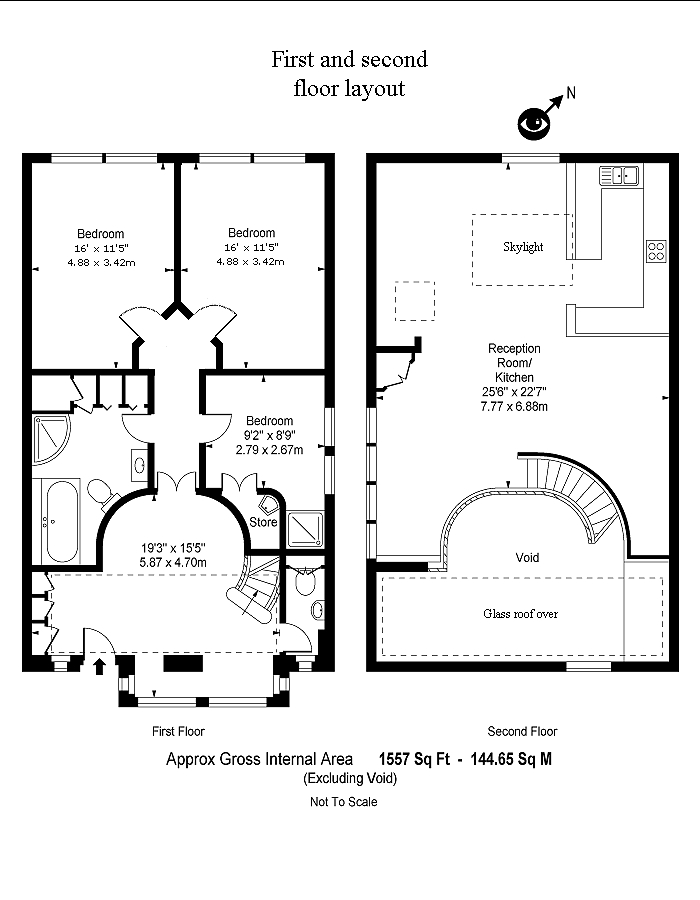This diagram is a detailed floor plan of a two-story house, showcasing the layout of both the first and second floors. The first floor plan is on the left side of the diagram, while the second floor layout is on the right. 

At the center of the diagram, a black circle with a white, eye-like cutout and an arrow pointing upwards to the 2 o'clock position indicates the house's orientation, with the arrow marking the northern direction.

**First Floor:**
- **Entrance Hall:** At the front of the building is the main entrance, leading into a spacious entrance hall measuring approximately 19 feet by 15 feet.
- **Staircase:** A sweeping staircase is positioned on the right side of the entrance hall.
- **Corridor:** There’s a corridor extending from the entrance hall. 
  - **Bedroom:** On the right, this corridor leads to a bedroom which includes its own shower and a small storeroom.
  - **Bathroom:** Opposite the bedroom, on the left side of the corridor, is a full bathroom equipped with a shower, basin, toilet, and bath.
  - **Additional Bedrooms:** Further along the corridor, there are two bedrooms, each measuring around 16 feet by 11 feet 5 inches.

**Second Floor:**
- **Balcony:** The staircase from the first floor leads up to a balcony area that overlooks the entrance hall below.
- **Open Plan Reception and Kitchen:** The second floor features a large, open-plan reception room combined with a kitchen area, which spans roughly 25.5 feet by 22.5 feet.
- **Skylight:** A skylight is also present, providing ample natural light to the spacious open area.

This detailed layout provides a comprehensive overview of the house’s structure, from the sizable entrance hall and well-distributed rooms on the first floor to the expansive open-plan living space on the second floor.